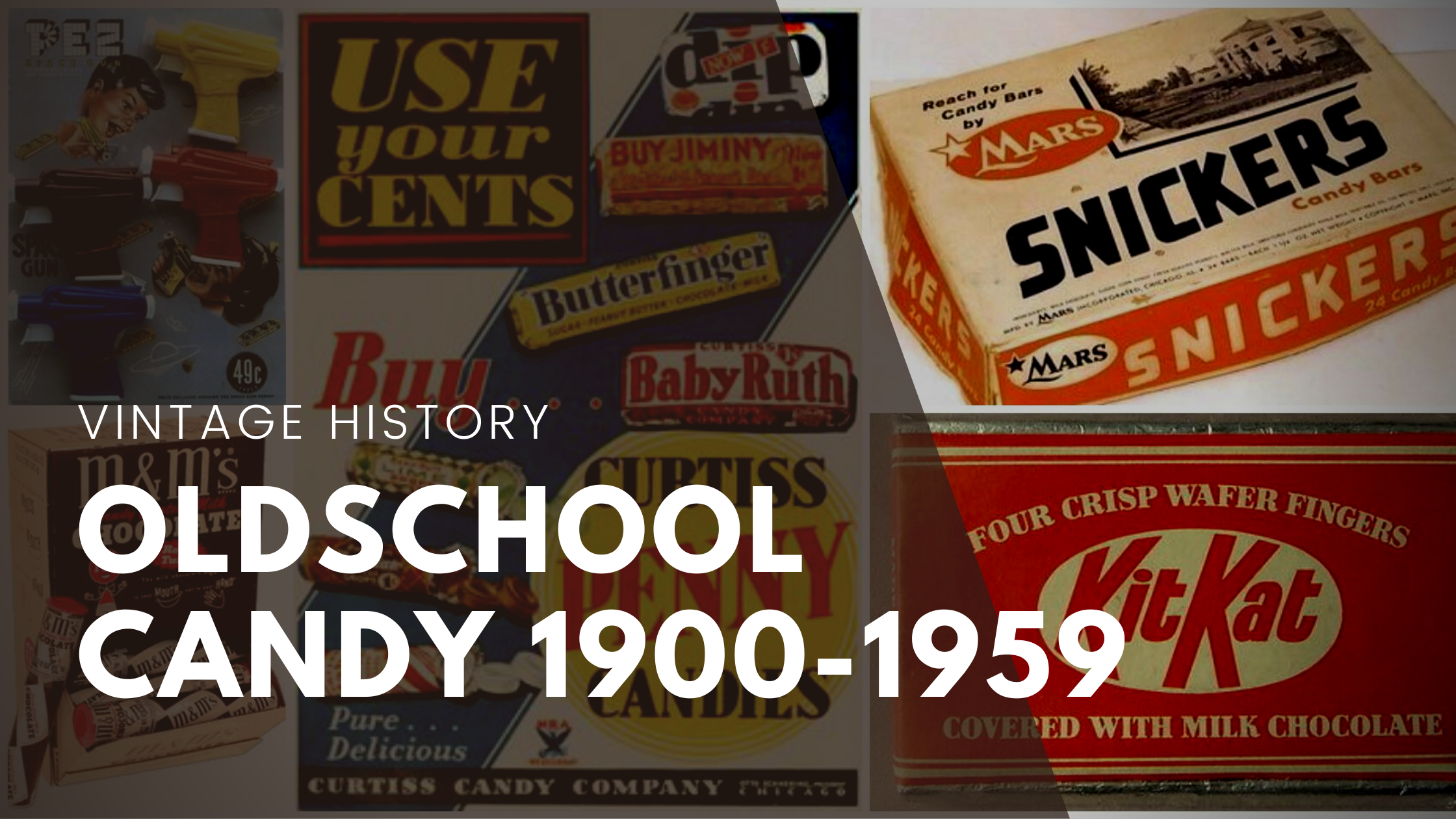The image is a wider-than-tall, vintage-themed collection of old-school candy advertisements from 1900 to 1959, set against a shaded background. The shading starts from about 60% down from the top left corner and runs diagonally to approximately the 70% point along the bottom. The left two-thirds of the image are notably shaded, emphasizing the contrast with the brighter right section. White text across the image proclaims "Vintage History Old-School Candy 1900 to 1959."

The collage features six different candy ads, arranged in two rows of three. In the top left, Pez dispensers in various colors (red, yellow, black, and blue) are displayed. Next to it, an ad reads "Use Your Sense," showcasing Butterfinger, Baby Ruth, and By Jimmies. At the top right is a prominent Mars Snickers candy bar ad. On the bottom left, M&Ms are featured, followed by Curtis Penny Candies in the center. Lastly, the bottom right showcases the Kit Kat logo with the description "Four Crisp Wafer Fingers Covered with Milk Chocolate." Each candy ad reflects the design and branding of its era, creating a nostalgic tableau of mid-20th-century sweets.